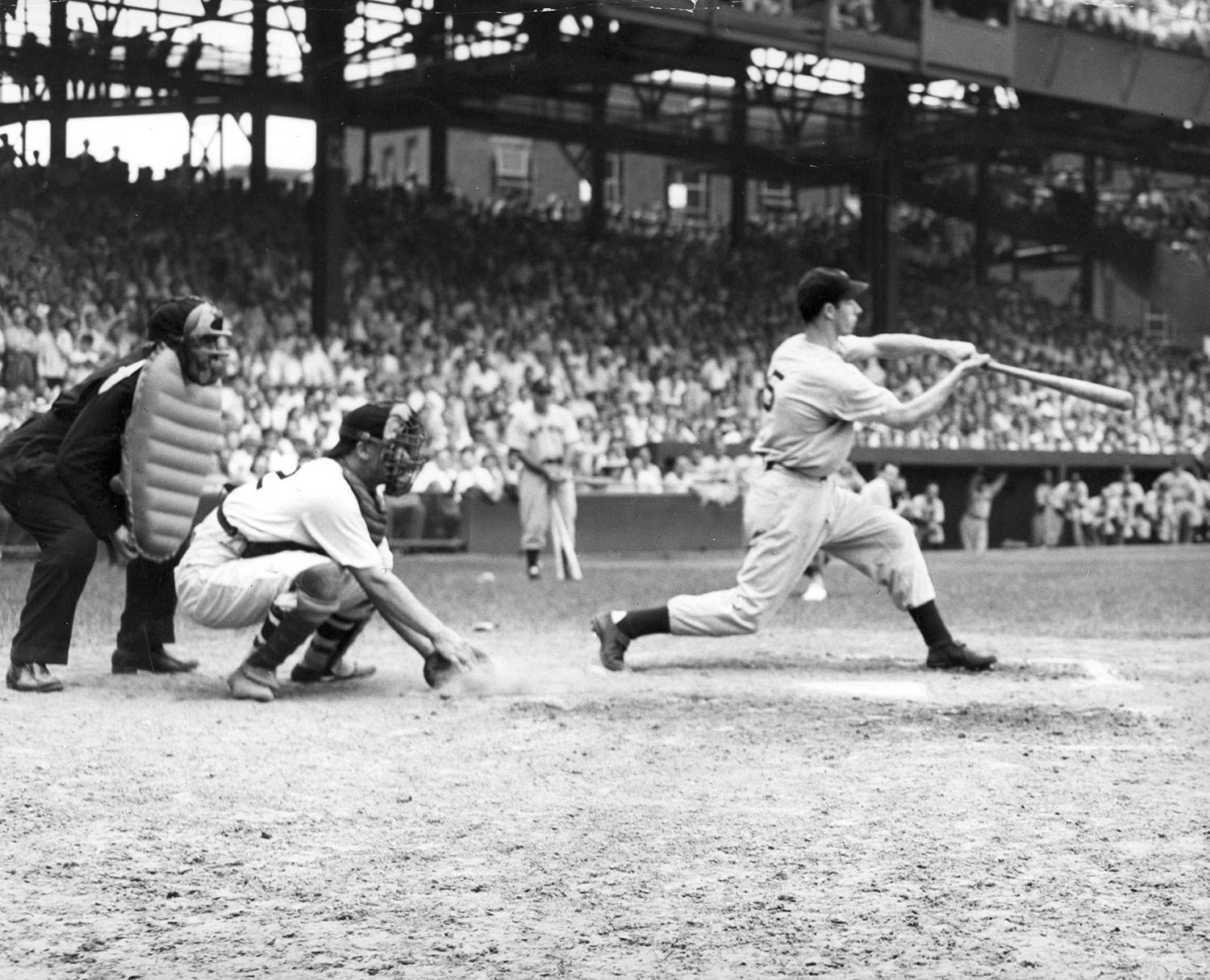The black-and-white image captures a historical moment from a baseball game, likely from the 1920s to 1940s, as suggested by the old-style uniforms. At the center of the scene, a baseball player stands at home plate, caught mid-swing with his bat in motion. Despite his effort, evidence suggests he missed the ball as the catcher, dressed in a white outfit with a mask, has his glove close to the ground, seemingly ready to catch the ball. Behind the catcher, the umpire in padded gear and a dark outfit is hunched down, intently watching the play. The surroundings indicate a lively game-day atmosphere; the stands in the background are filled with spectators, many dressed in white. A steel structure, possibly a bridge or walkway, runs along the top of the image, adding to the historic feel of the scene. An additional player is visible, poised to bat next. The field is a mix of dirt and grass, typical of the ballparks from that era. The photograph vividly encapsulates a moment of anticipation and energy in early 20th-century baseball.